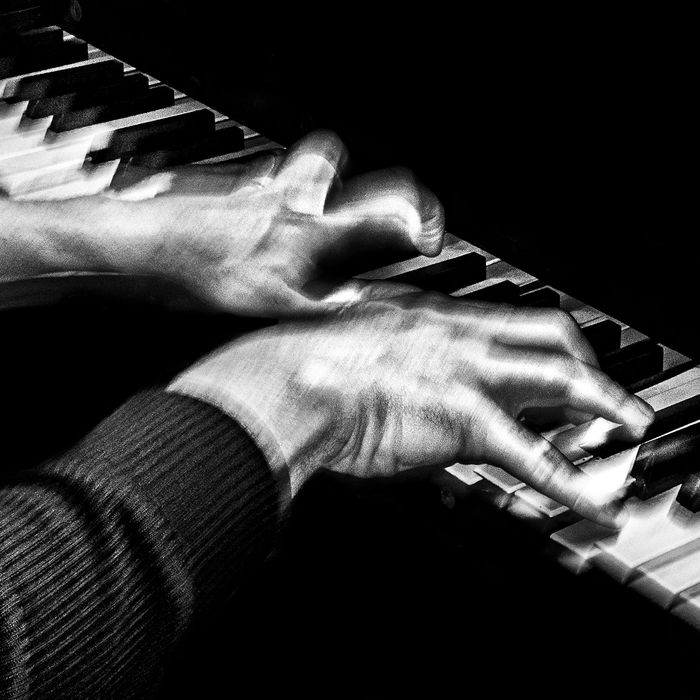The image is an artistic black and white rendering of a person playing a piano, with the focus on their hands and the piano keys. The square-shaped image has a primarily black background, enriched with shades of gray, giving it a hand-drawn or possibly digitally animated look. The scene captures the detail of a long-sleeve sweater worn by the pianist, with their left hand positioned in a claw-like grip pressing multiple shiny white keys, while the right hand is similarly poised. The keys span diagonally from the top left to the bottom right of the image. The shading on the hands highlights their light color and tension, adding to the intense atmosphere. The artistic rendering, slightly blurry and out of focus, suggests a sense of motion or speed in the playing. The piano's surrounding frame is black, contrasting starkly with the keys, completing the monochromatic, richly detailed composition.